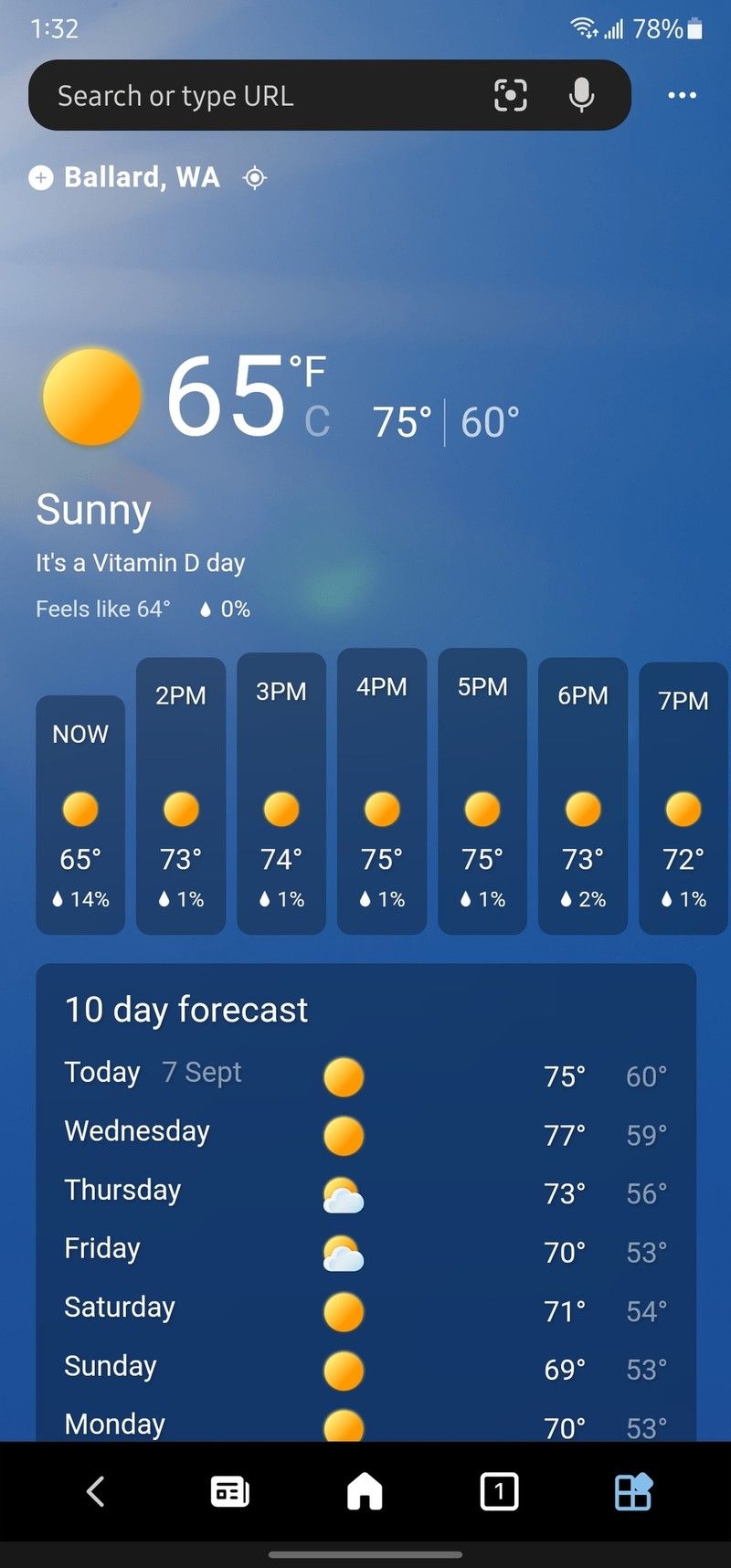Screenshot of a cell phone display taken at 1:32 (either a.m. or p.m.), showcasing the phone's status and the weather forecast for Ballard, Washington. The phone has 78% battery left, is connected to Wi-Fi, and shows full cellular signal bars. At the top of the screen, there's a search bar with options to search or type a URL, and includes icons for image search, voice input, and a menu.

Below the search bar, the location is given as Ballard, Washington, with the current temperature being 65°F. The high for the day is expected to reach 75°F, and the low will be 60°F. The weather summary states it is sunny and notes, "It's a vitamin D day," with the temperature feeling like 64°F and a 0% chance of precipitation for the current time. 

The detailed hourly forecast is as follows:
- 2 p.m.: 73°F with a 1% chance of precipitation
- 3 p.m.: 74°F with a 1% chance of precipitation
- 4 p.m.: 75°F with a 1% chance of precipitation
- 5 p.m.: 75°F with a 1% chance of precipitation
- 6 p.m.: 73°F with a 2% chance of precipitation
- 7 p.m.: 72°F with a 1% chance of precipitation

Below the hourly forecast, a 10-day weather forecast begins with today, September 7th, showing a high of 75°F and a low of 60°F. The upcoming days include:
- Wednesday: Sunny with a high of 77°F and a low of 59°F
- Thursday: Partly cloudy with a high of 73°F and a low of 56°F
- Friday: Partly cloudy with a high of 70°F and a low of 53°F